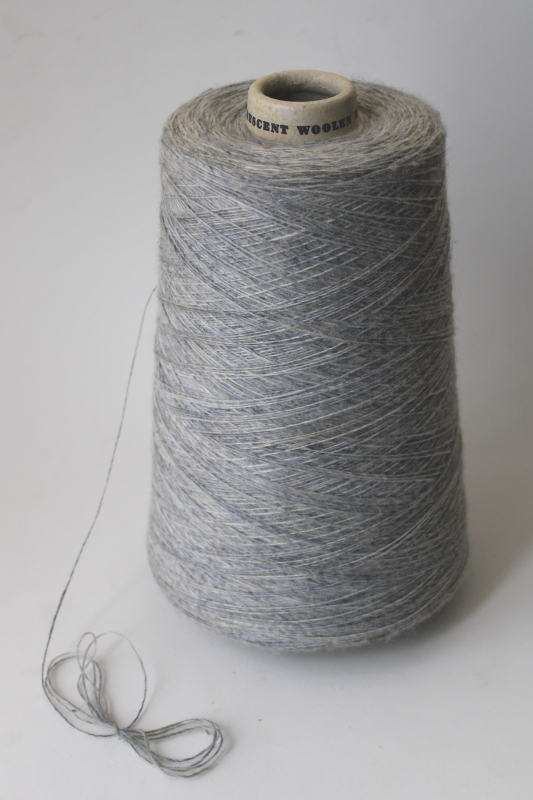A detailed photograph showcases a large, conical spool of gray thread. The spool has a slightly whiter base, giving a contrast to the primarily gray color of the thread. An end of the thread protrudes from the mostly full spool, creating a small, neat bundle where it has been folded over and tied delicately. The label on the spool appears to read something akin to "Sent Wool," hinting at either the brand or the type of thread. The entire scene is set against a similarly gray background, enhancing the monochromatic theme and drawing focus to the subtle details of the spool and thread.